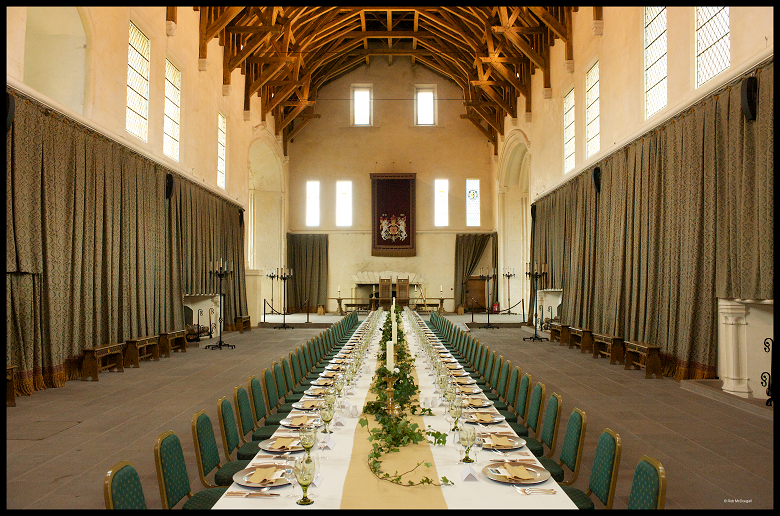The image depicts the interior of an expansive, royal banquet hall with striking features reminiscent of a church, accentuated by the high, curved ceiling supported by large wooden beams. The long, narrow room is bathed in light from numerous tall windows that line the upper portions of the left and right walls, as well as the back wall, which features an array of six windows—two near the ceiling and four aligned with the others. The walls, painted in an off-white hue, are adorned with lush green curtains from midway to the floor and are complemented by benches positioned beneath the windows.

Dominating the center of the hall is an elongated banquet table extending from the back to the front of the room. This table is draped in a white tablecloth, with a burlap-colored table runner adorned with decorative plants and white candles in gold candlestick holders. The table is surrounded by numerous green cushioned chairs with gold trim, potentially seating between 20 to 25 guests on each side, and two larger chairs at one end, suggesting places of honor.

The room also features two archways on either side at the back, draped with curtains, and a small stage covered in white. A notable tapestry hangs prominently on the back wall, flanked by additional windows, creating a sense of grandeur and history within this stately dining area.